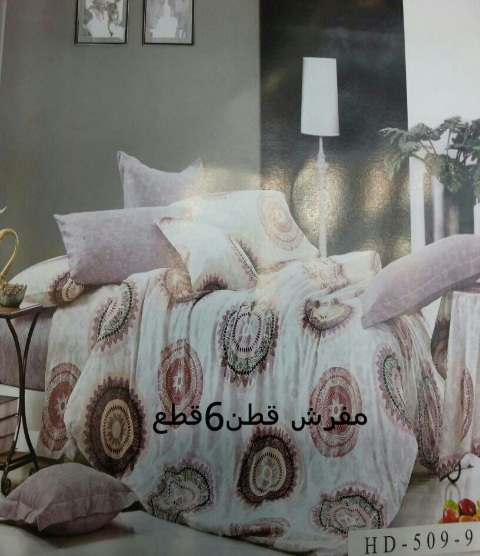A photograph captures a printout of a page from a furniture catalog, showcasing a bedroom setup centered around a bed with an ornate white bedspread. The bedspread, adorned with intricate circular patterns reminiscent of doilies and dreamcatchers, features an array of colors, including dark maroon, dark brown with yellow, dark black, and orange. These circular designs are scattered across the textile, giving it a detailed and elegant look. Multiple pillows rest atop the bed, some matching the bedspread's ornate pattern, and others in plain mauve and gray. 

The room's backdrop includes a smooth gray wall with black accents, possibly a door, and a white wall on the right side. The wall behind the bed also displays two framed photos with black frames. A small black side table with a black steel base and a rectangular brown wooden top is positioned to the left of the bed. Additionally, there's a white carpet in front of the bed and a light purple pillow on the ground, further adding to the room's layered decor. Text elements in black Arabic lettering stretch across the bottom of the photo, and in the bottom right corner, the identifier "HD-509-9" is prominently displayed. Reflections of light are visible on the printed paper due to the photograph's lighting.